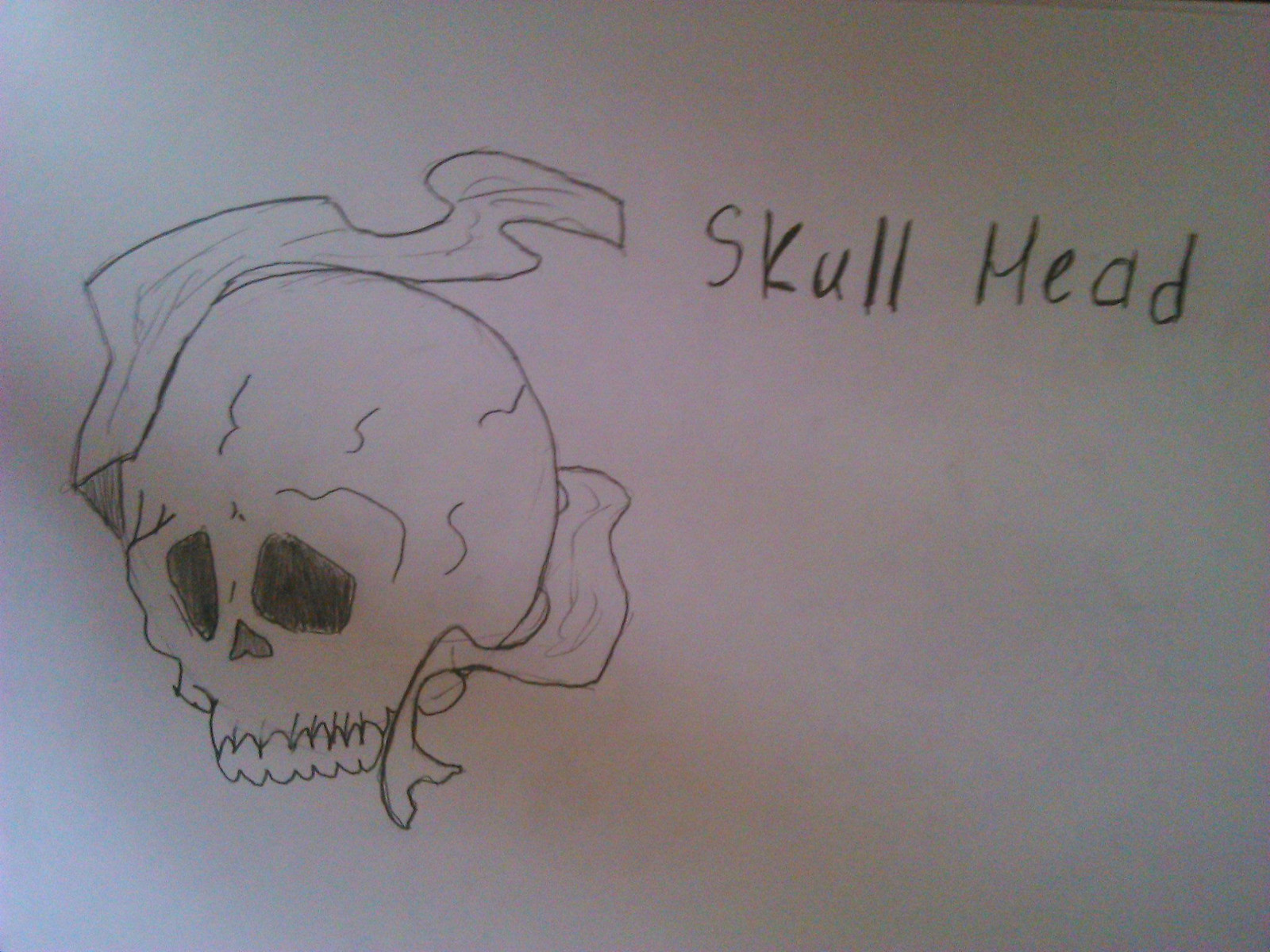This detailed pencil drawing, set against a stark white piece of paper, features a skull without its lower jaw positioned on the left side. The skull, while anatomically incorrect with misaligned features such as the eye sockets and upper jaw, and lacking ear holes, is intricately rendered. The top and back of the skull, as well as the ear socket, are draped with cloth that adds a sense of texture and depth to the artwork. Emanating from the sides of the skull are squiggly lines, reminiscent of smoke, adding a dynamic element to the piece. To the right of the drawing, near the top, the words "Skull Mead," written in pencil and having a slight error ("Skull Head" misinterpreted as "Skull Mead"), juxtapose against an otherwise vast expanse of white space, emphasizing the central morbidity of the skull. Despite its anatomical inaccuracies, the drawing conveys a compelling visual narrative, showcasing the artist's skill in creating a dramatic, monochromatic composition.